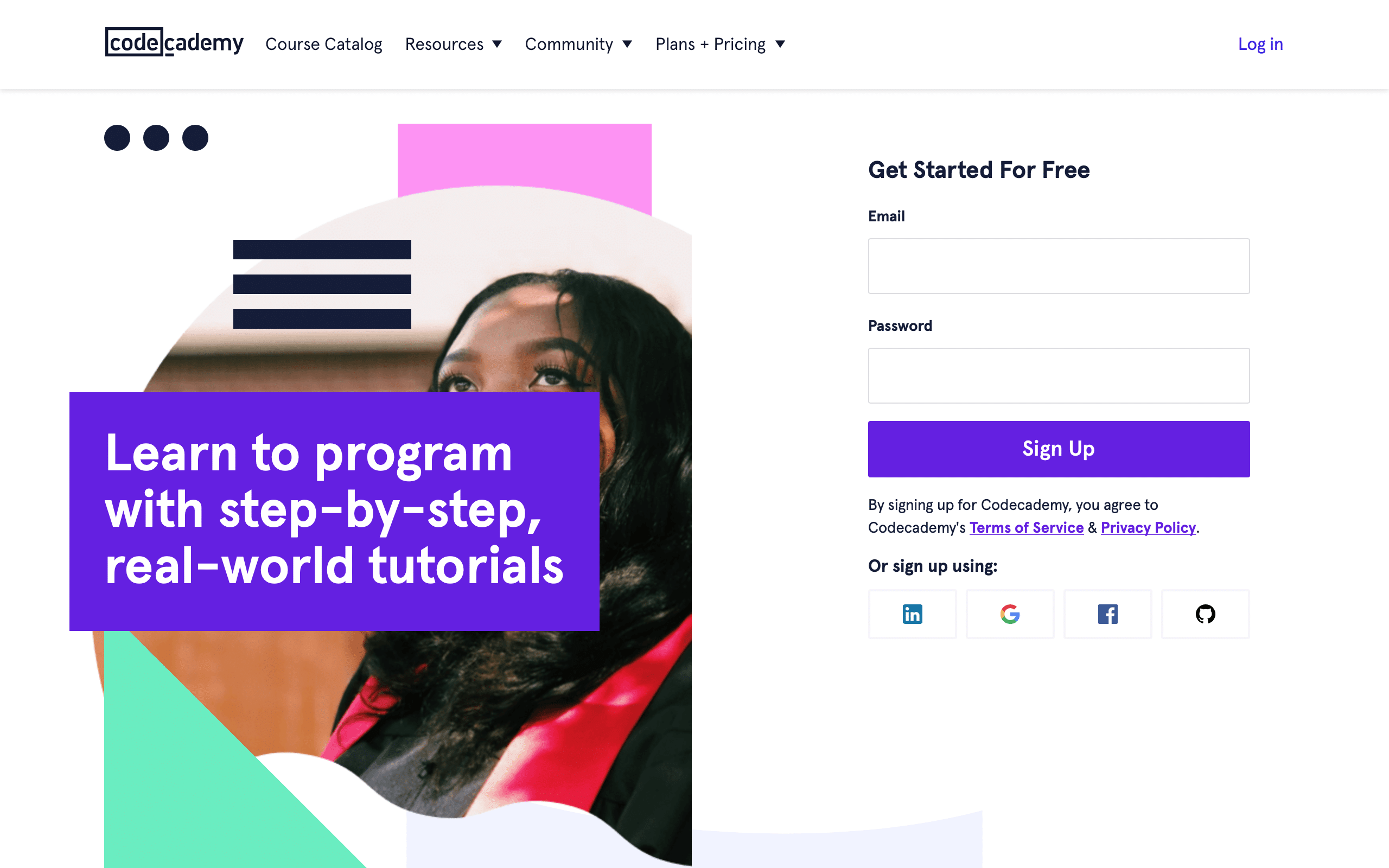The image features a clean, white background with a prominent header at the top displaying the text "Code Academy" in blue, with the word "Code" enclosed in a small rectangular box. Below this, there is a navigation bar offering links titled "Course Catalog," "Resources," "Community," and "Plans and Pricing," each accompanied by a drop-down menu. To the right of these links, there are options for "Login" and a row of three black dots followed by a short horizontal line.

Prominently displayed below the header is a central section highlighted by a half-round gray background with a purple square overlaying it. Adorning the background are three black horizontal lines, intersected by the purple box. In this section, a headline in bold text reads, "Learn to Program with Step-by-Step Real World Tutorials." To the left, there is an image of a girl looking upwards, which adds a human element to the promotional material. A large blue triangle rests at the bottom left corner of this section.

On the right side of the central section, a call-to-action reads, "Get Started for Free," positioned above a form asking for an email address and password. Just below these input fields is a purple sign-up button. In smaller text below the button, users are informed that by signing up, they agree to Code Academy's Terms of Service and Privacy Policy. Additionally, there are options to sign up using third-party services such as Google or Facebook.